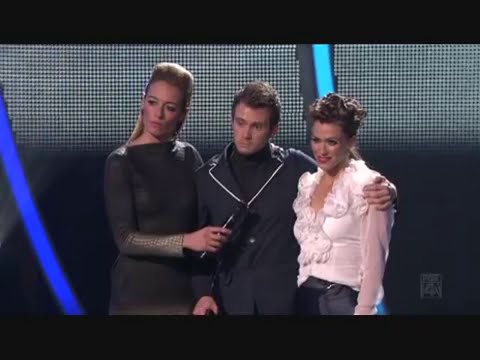The image depicts a scene from what appears to be a television show, possibly a game show or reality show. Three people are standing on a stage with a backdrop featuring blue fluorescent lines and a black, spotted background. 

In the center is a man with brown hair, clothed entirely in black, including a jacket with white piping on the collar and a black turtleneck. He has his arm around a woman to his right. This woman has brown hair styled up and is wearing a white floral-patterned shirt. She is smiling and appears to be looking at something or someone off-camera, possibly judges. 

To the man's left is another woman with tall, blonde hair placed down in the back, wearing a black and gray dress, and holding a microphone in front of the man. She looks like an announcer, poised to speak. 

In addition to the people, the scene includes a black border at the top and bottom of the screen, with a barely discernible logo in the lower corners, and a blue line running along the left side of the screen.